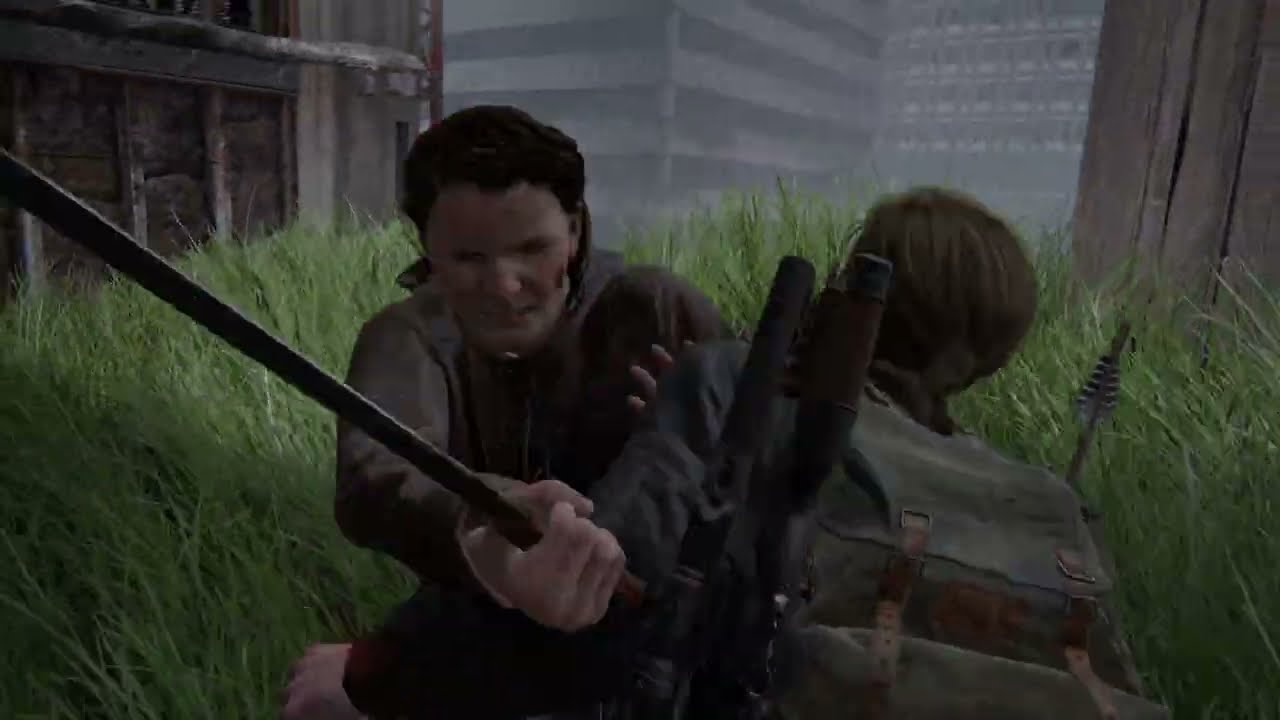The image depicts a slightly pixelated and cartoonish screenshot from a video game, featuring two characters engaged in a tense confrontation in a grassy field with various buildings in the background. The central figure, a man with dark black-brown hair, is brandishing a sword or metal rod and appears to be about to attack. Opposite him, a younger woman with medium-brown hair, seen from the back, is sporting an olive green backpack with noticeable items protruding from both sides, likely weapons. The woman, who seems to be wearing outdoor clothes, is attempting to fend off the man by grabbing his shoulder and the pole in her arm, which might be a spear or stake. Neither character is wearing a helmet. The setting features long grass in the foreground and a mix of wooden structures and skyscrapers, some of which appear foggy, in the background.